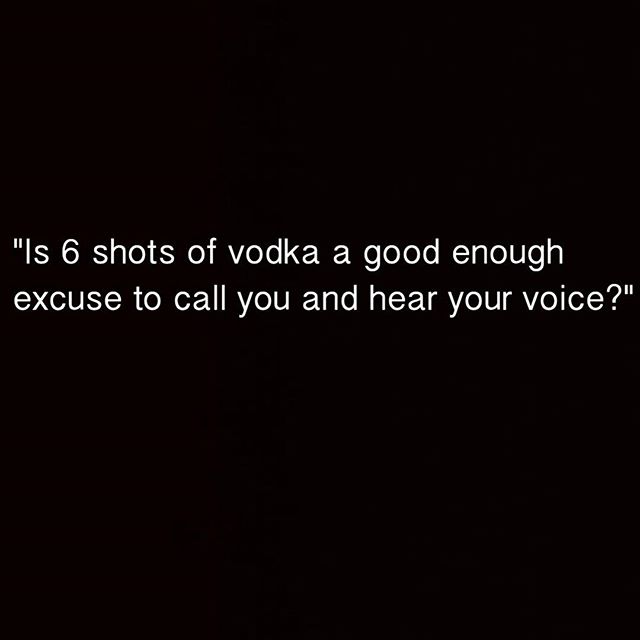The image features a solid black square background with white text at the center, slightly above the middle of the square. The text is presented in two lines using a clean, sans-serif font, likely Arial. The quote, enclosed in quotation marks, is arranged as follows: the first line reads, "Is six shots of vodka a good enough," and the second line continues with, "excuse to call you and hear your voice?" The text is centered and the quotation is complete with proper English punctuation, including the question mark inside the closing quotation mark.